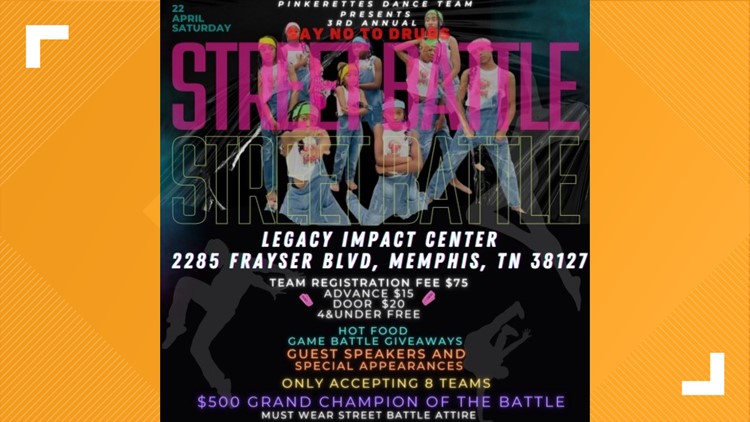This image features a detailed flyer advertising the third annual "Say No To Drugs" Street Battle, presented by Pinkarette's Dance Team. The flyer predominantly has a striking black background with golden-yellow borders on the left and right sides. At the top left and bottom right corners, there are white L-shaped designs that resemble incomplete squares.

The main content in the center of the flyer promotes the event, with "Street Battle" prominently displayed in vibrant colors — the top "Street Battle" text is pinkish-purple, while the bottom text is semi-transparent. Positioned behind this text are silhouettes of dancers striking dynamic poses, adding an energetic feel to the advertisement. 

The flyer provides detailed information about the event. It is scheduled for the 22nd of April, a Saturday, and will take place at the Legacy Impact Center, located at 2285 Fraser Boulevard in Memphis, Tennessee, 38127. The team registration fee is $75, with advanced tickets available or $15 at the door, going up to $20 on the day of the event. Children aged four and under can attend for free. Additionally, attendees can expect hot food, game battle giveaways, guest speakers, and special appearances, with the competition's grand champion receiving a $500 prize.

At the very bottom of the flyer, various promotional elements are listed in different colors, including white, green, orange, and purple texts, ensuring key details stand out. The flyer also portrays logos of dancing silhouettes, reinforcing the dance battle theme. Overall, the design meticulously balances informative content with eye-catching visuals to attract participants and attendees to the event.